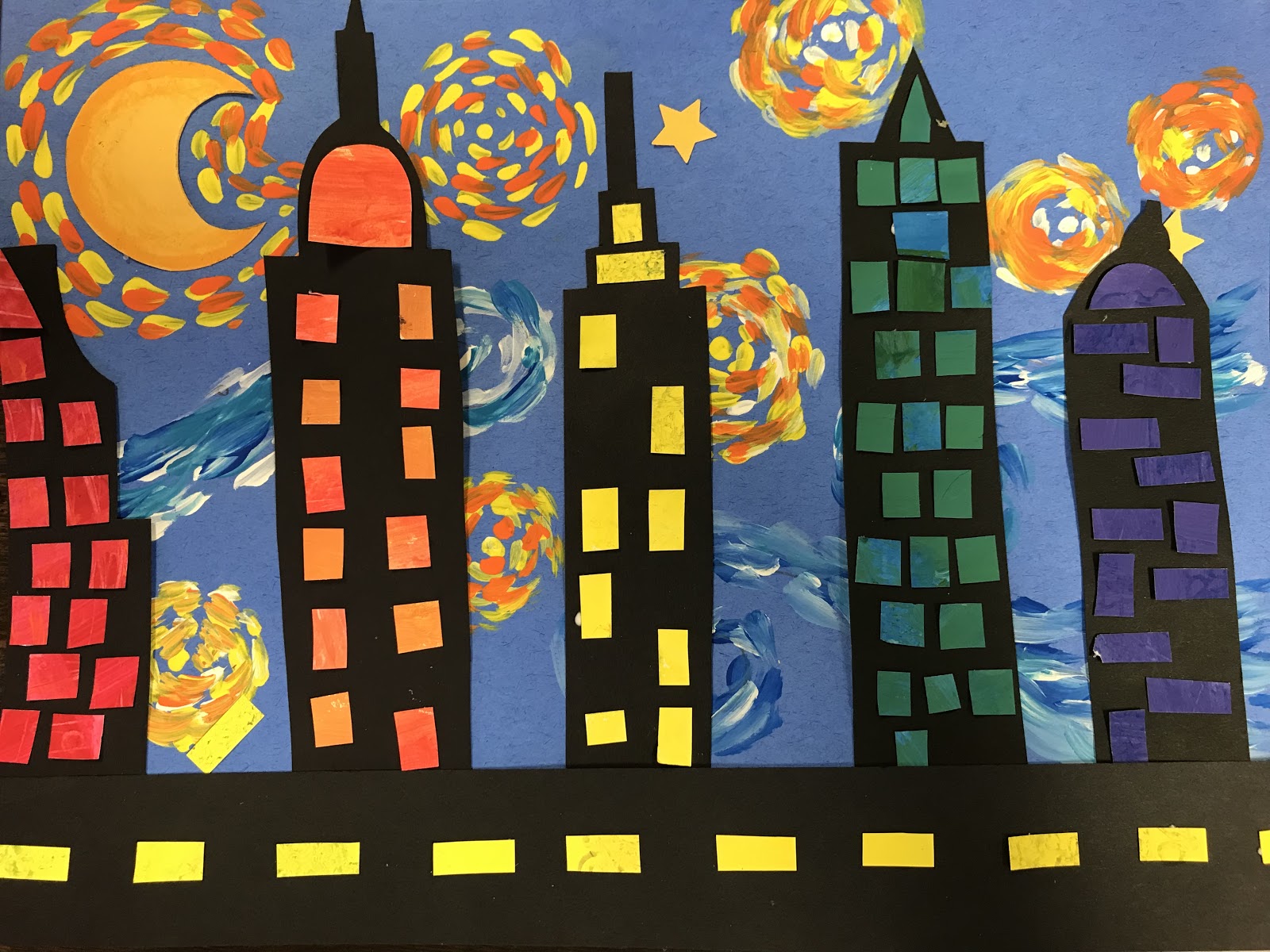A photograph captures a charming, childlike artwork depicting a whimsical cityscape. The artwork's background is a blue canvas, reminiscent of Van Gogh's Starry Night, adorned with swirling colors in oranges and blues symbolizing wind and stars. Among these swirls, a single yellow star and an orange crescent moon with dotted patterns stand out. The foreground presents five black skyscrapers with vibrantly colored windows made from cut-out construction paper: the leftmost building with red windows, followed by ones with orange, yellow, green, and purple windows respectively. These buildings rest atop a black road, complete with yellow dashed lines made from paper, forming a makeshift highway. The overall composition, with its crude cut-outs and vibrant color scheme, exudes an innocent, amateurish charm, likely intended to mimic the artistic expressions of a child using simple materials.